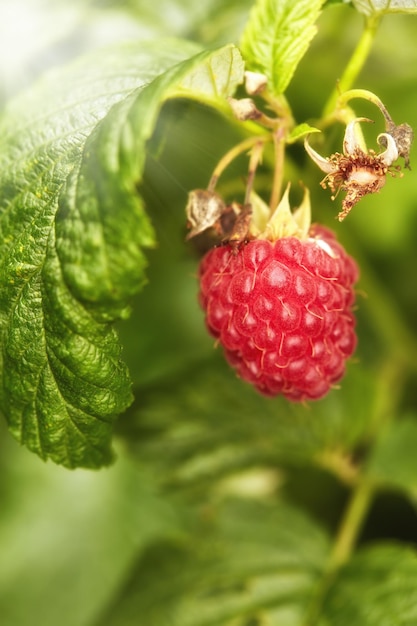In this detailed close-up image, a single, vibrant red raspberry hangs from a stem surrounded by lush green, slightly blurry leaves that form the backdrop. The raspberry is prominently featured in the top left section of the image, displaying a rich, dark red hue with delicate hair-like structures reminiscent of corn silk. The plant’s leaves are fresh green, contrasting with the reddish-brown ridges of the stem from which a raspberry has likely been picked, possibly eaten by an animal or a person. The berry itself has an intricate pattern of circular bulbs, adding texture and detail. The depth of field is shallow, concentrating the viewer's attention on the beautifully lit raspberry, while the sun highlights the scene with a bright spot in the upper left corner. The image is taken outdoors, with a natural setting that emphasizes the vividness of the raspberry against the softer, green foliage in the blurred background. No insects or other creatures are visible, making the raspberry the undisputed focal point of the composition.